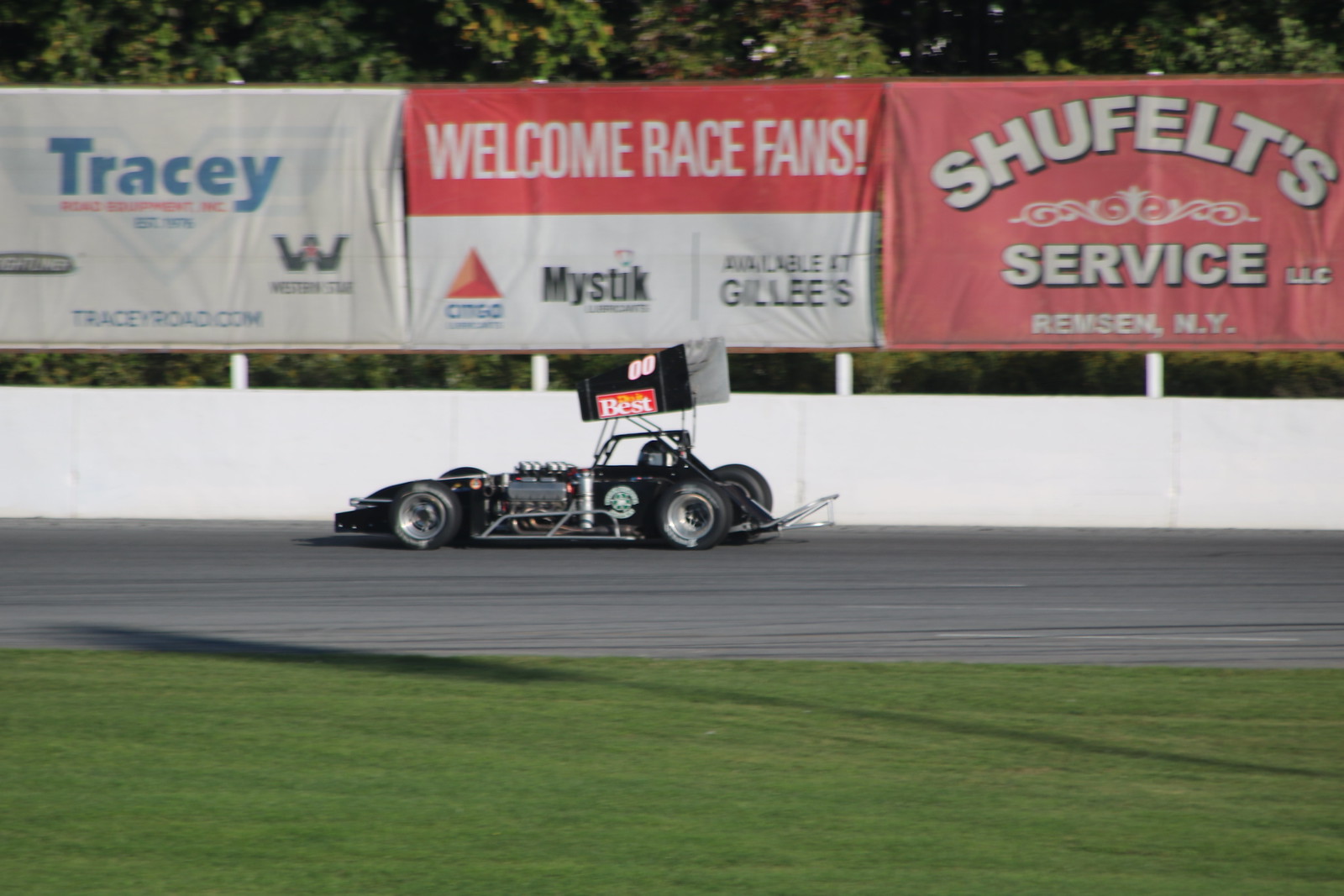The image captures a dynamic scene of a black race car, numbered 00, speeding from right to left on a grey racetrack. In the foreground at the bottom of the image lies a grassy infield, giving way to the racecourse surface above it. The car, sleek and low to the ground with prominent silver features including a sizable exposed engine and bumpers, showcases a black spoiler and what appears to be a roll bar. You can see the driver, clad in a black helmet, positioned inside. Behind the car is a short white wall, above which numerous billboards are mounted on white poles. The billboard on the far left reads "Tracy Road Equipment" in blue text, the center one welcomes race fans with additional mentions of sponsors like Citgo, Mystique, and Gillies, and the far-right billboard advertises "Shuffle Felt Service" on a red background, noting Remsen, NY. Beyond the advertising signs, a line of trees sets the backdrop for this energetic racing scene.